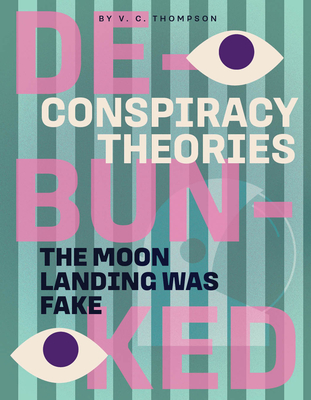This detailed book cover features a striking striped background consisting of alternating vertical stripes in two shades of green: a darker green and a lighter, mint green. The title, "Debunked," is prominently displayed in vibrant pink lettering, with the subtitle "Conspiracy Theories" in white text directly below it. Towards the bottom, the phrase "The Moon Landing Was Fake" is boldly written in black letters. The book is authored by V.C. Thompson, as indicated at the top of the cover. Adding to its unique design, there are two illustrated eyes with white backgrounds and purple pupils, one positioned at the top right and the other at the bottom left of the cover. This eye-catching and intricately designed cover is both intriguing and visually appealing, effectively drawing attention with its colorful and bold elements.